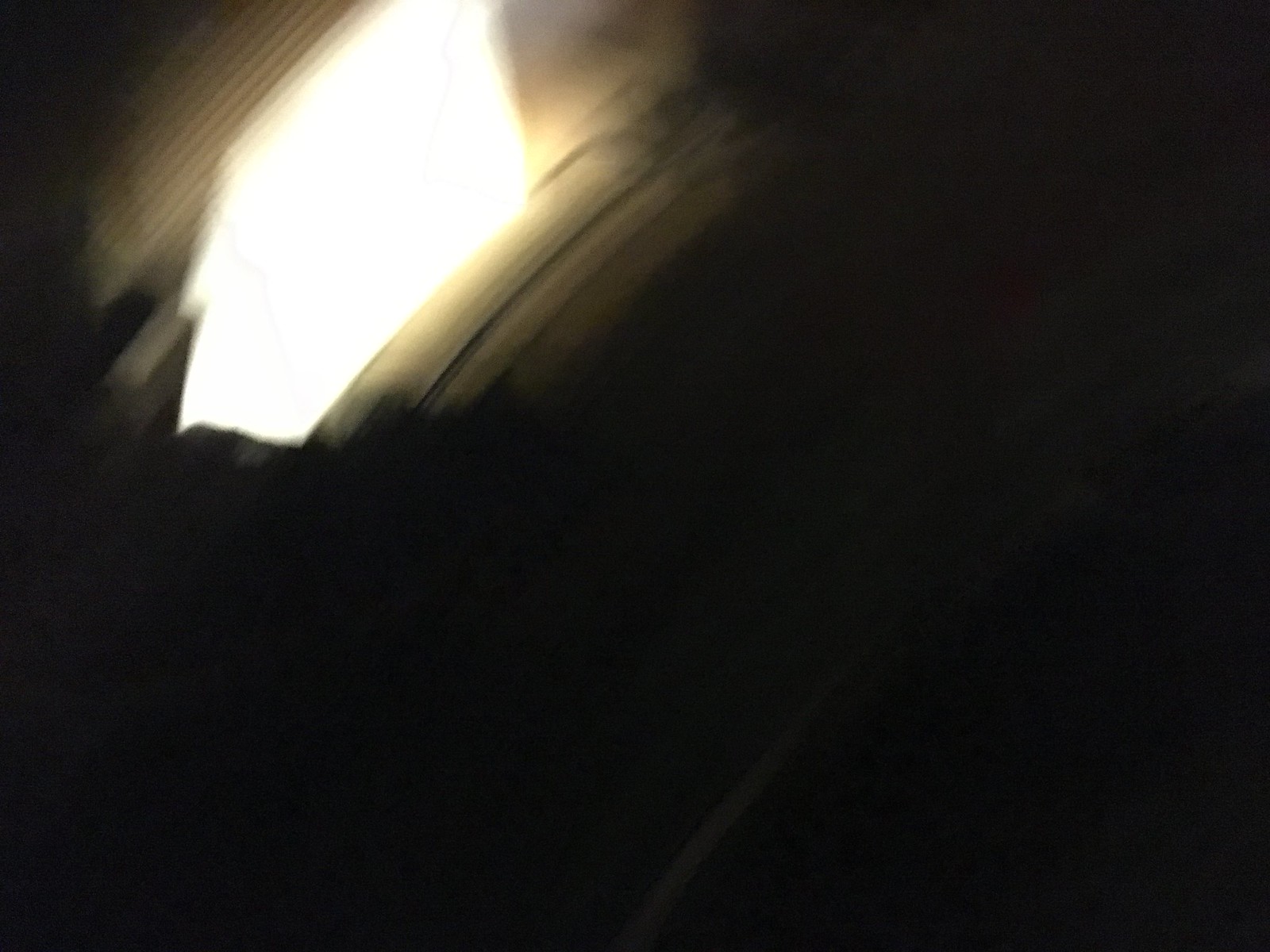This image is a blurred photograph, predominantly dark and out of focus. The majority of the picture is obscured in blackness, leaving little to discern. However, the upper left-hand corner features a bright rectangular block of white light, possibly from a vehicle's headlights or a lighting fixture. This light radiates a tan glow, creating some grayish stripes and shapes against the surrounding black. Hints of possible roadside elements or trees are vaguely visible on the outskirts, along with suggestions of a vehicle’s silhouette. The overall effect is one of motion blur, indicating the camera was likely unstable when the photo was taken and resulting in an image that is difficult to interpret.